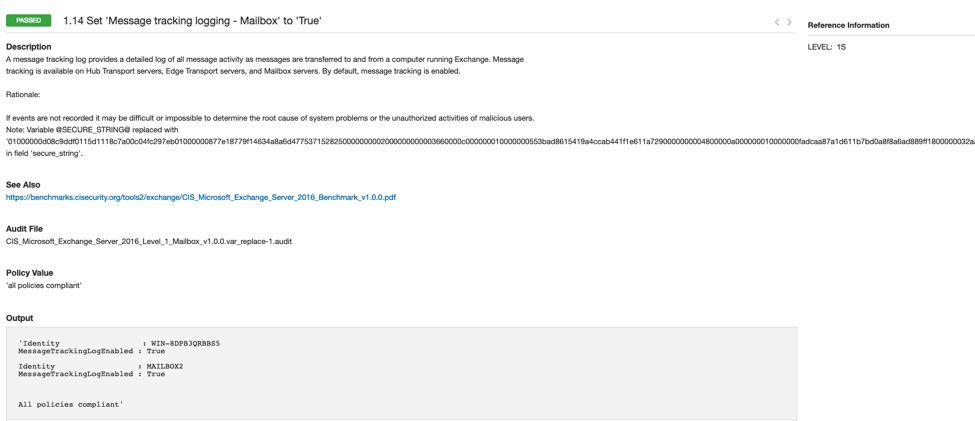In this image, we see a detailed information page related to message tracking logs in a messaging system. At the top of the page, the header reads "1.14 Message Tracking Log." The section provides a comprehensive explanation of message tracking, which logs all message activities as they are transmitted to and from a computer running an Exchange server. Message tracking is applicable to Hub Transport servers, Edge Transport servers, and Mailbox servers, and is enabled by default.

The rationale given emphasizes the importance of recording these events, stating that without message tracking, it could be challenging or impossible to identify the root cause of system issues or unauthorized activities conducted by malicious users.

Additionally, there are notes at the end of the page signifying that variables at the 6th string have been replaced with the phrase "see also." A link is provided under the "See Also" section for further reference.